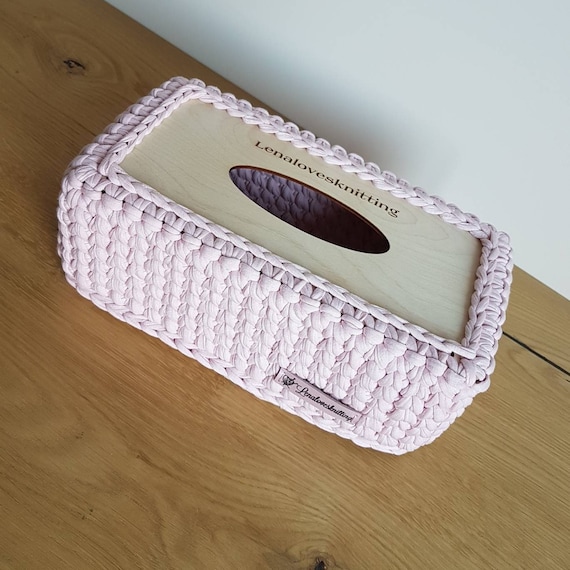This image captures a detailed view of a pastel pink crocheted tissue box cover, designed to encase a standard cardboard tissue box. The cover features a light wood or laminate top with an oval opening, through which tissues can be accessed. The top of the cover is adorned with the phrase "Lena loves knitting," suggesting it might be handmade or a product of a small business. The phrase appears to be either burned or printed in brown on the wooden section. There is also a cloth label on the side of the cover that repeats the same phrase, "Lena loves knitting." The entire setup is situated on a light brown wooden table with a cream-colored wall in the background. The photograph is taken at a slight diagonal angle, adding a dynamic touch to the composition.